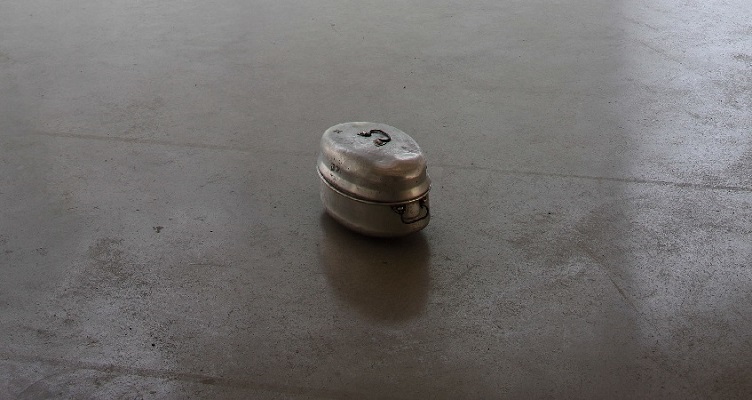The image showcases a weathered, oval-shaped roasting pot with a shiny, chrome stainless steel finish, placed in the center of a textured, cobalt gray floor. The surface, likely made of concrete or hard metal, features some specks of dirt and discernible lines of demarcation, positioned both horizontally and vertically. The pot itself is small and equipped with a lid that has a handle on top, along with one visible side handle on the right, suggesting a matching handle on the left. The pot appears to be well-used, with visible dents and possibly a faint number on its side. The overall color scheme of the image includes various shades of gray, black, silver, and a touch of white, giving the scene a somewhat modern or abstract art feel. There are no organic elements present, emphasizing the stark, industrial ambiance of the photograph.